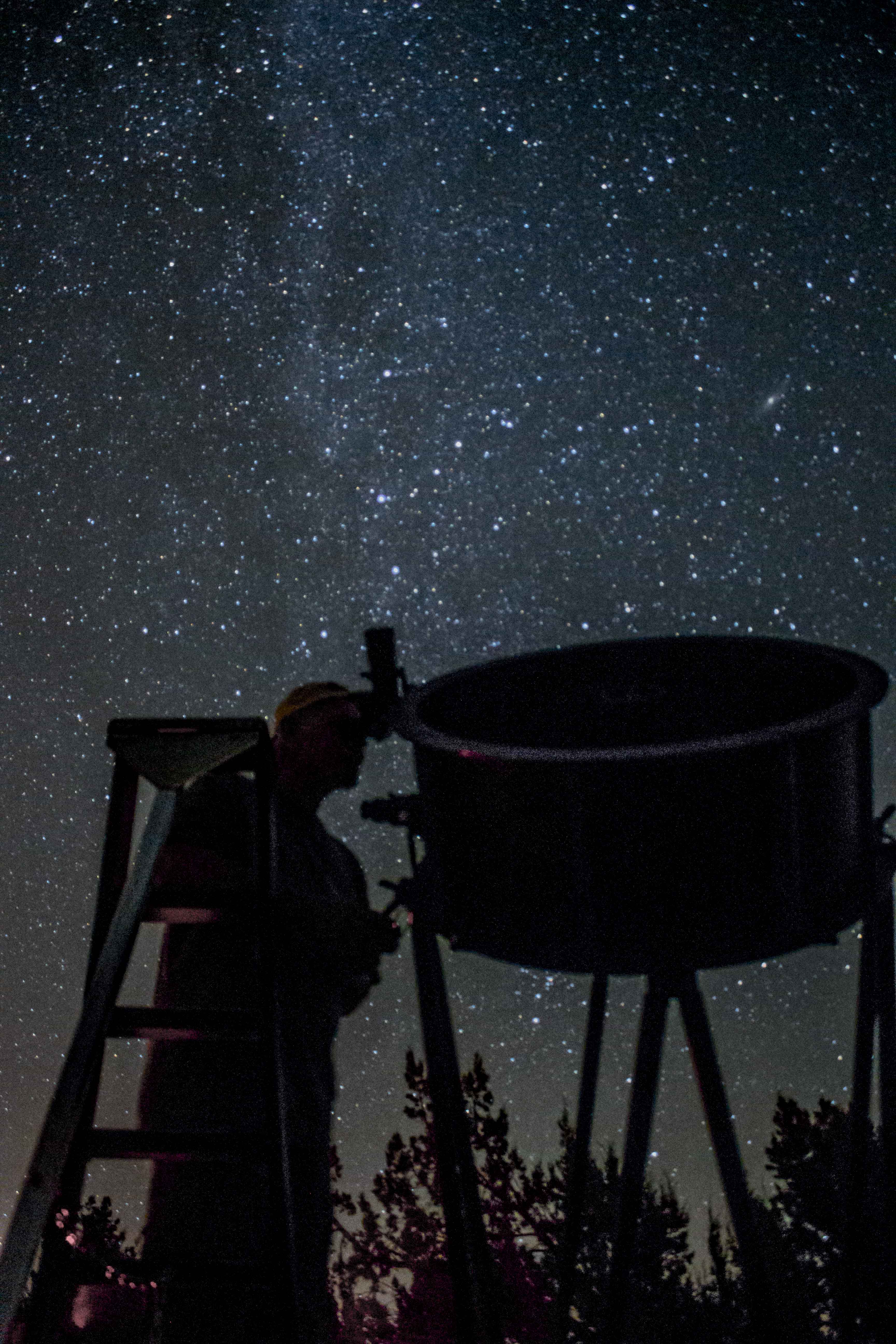In this evocative nighttime scene, a man dressed in dark clothing and a hat can be seen intently peering through the viewfinder of a large compound telescope. The telescope, a broad cylindrical structure approximately three feet in diameter and a foot and a half in depth, is supported by an intricate network of cross-hatched bars and elevated on sturdy legs. To reach the elevated viewfinder, the man stands on a ladder positioned at the left of the image. Surrounding this setup, the night sky stretches wide, densely populated with stars that create a mesmerizing backdrop. The landscape includes the faint silhouettes of treetops at the bottom of the scene, blending seamlessly with the starlit sky. The entire scene is bathed in hues of black, blue, white, and hints of grey and a slight purple, hinting at either a digitally enhanced photograph or a computer-generated image, capturing the serene and awe-inspiring beauty of a stargazer’s moment under the cosmos.